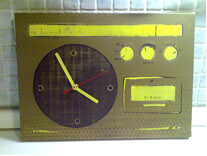The image depicts a photograph of a bronze-ish brown rectangular object, possibly a clock radio or an answering machine, displayed against a backdrop of small, light blue or silver-blue tiles. On the left side of the object, there is a large, black clock face with bright yellow hour and minute hands, a red second hand, and yellow circles at the 12, 3, 6, and 9 positions instead of numbers. The clock shows the time to be approximately 3:55. Across the top of the object is a yellow banner running almost its entire width. To the right of the clock face, there are three yellow circular knobs or buttons lined up horizontally, and below them is a yellow rectangular area that possibly could be a display or another function difficult to decipher due to the image’s small size. The entire scene appears to be brightly lit, highlighting the intricate details of the object and its surroundings.